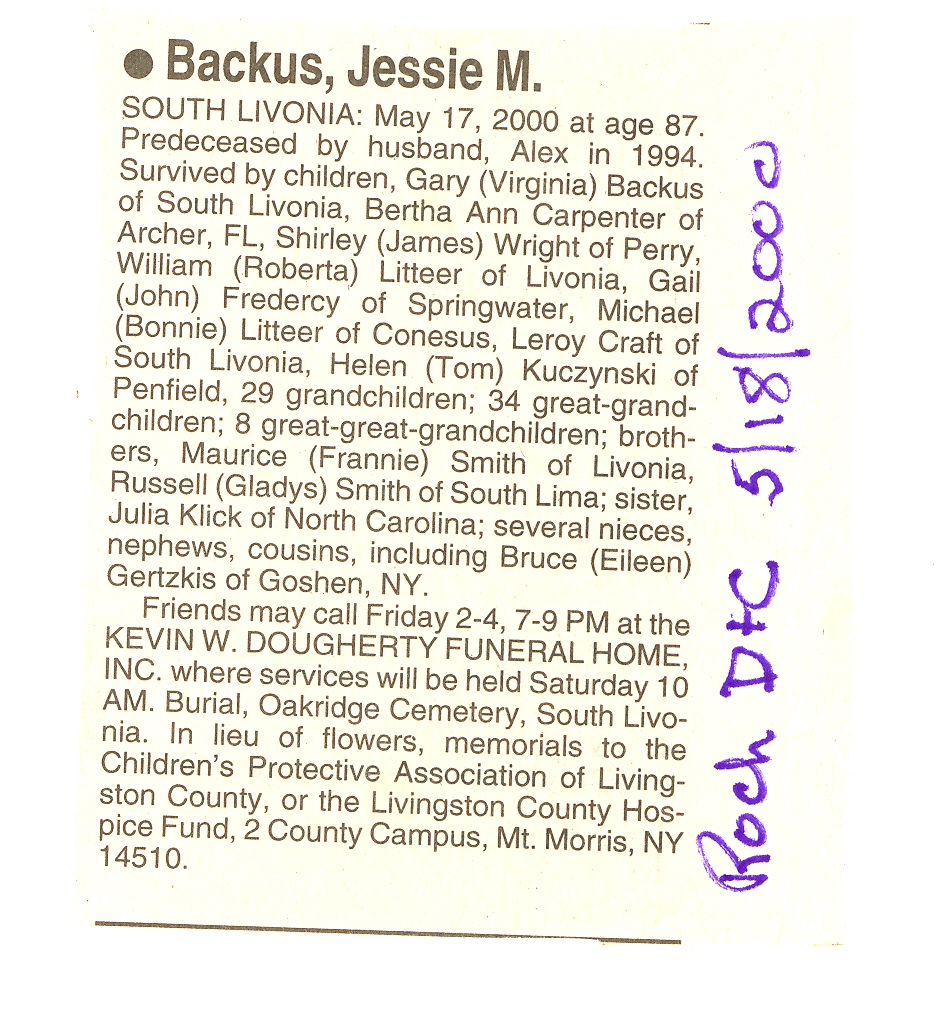The image depicts a faded newspaper clipping on a subtle white background with a faded black circle at the top. Handwritten in blue ink along the right side is "ROCH D+C 5/18/2000." The main text is an obituary for Jesse M. Bacchus, which reads:

"South Livonia, May 17, 2000, at age 87. Pre-deceased by husband Alex in 1994. Survived by children Gary Virginia Bacchus of South Livonia, Bertha Ann Carpenter of Archer, Florida, Shirley James Wright of Perry, William Roberta Latere of Livonia, Gail John Friderici of Springwater, Michael Bonnie Latere of Conesis, Leroy Craft of South Livonia, Helen Tom Kaczynski of Penfield; 29 grandchildren, 34 great-grandchildren, 8 great-great-grandchildren. Brothers: Maurice Franny Smith of Livonia, Russell Gladys Smith of South Lima; Sister: Julia Click of North Carolina; Several nieces, nephews, cousins, including Bruce Eileen Gertzkes of Goshen, New York. Friends may call Friday 2-4 p.m. and 7-9 p.m. at the Kevin W. Dougherty Funeral Home, Inc. Services will be held Saturday, 10 a.m., with burial at Oak Ridge Cemetery, South Livonia. In lieu of flowers, memorials may be made to the Children's Protective Association of Livingston County or the Livingston County Hospice Fund, 2 County Campus, Mount Morris, New York 14510."

The text captures the detailed lineage and funeral arrangements, commemorating the life and legacy of Jesse M. Bacchus.